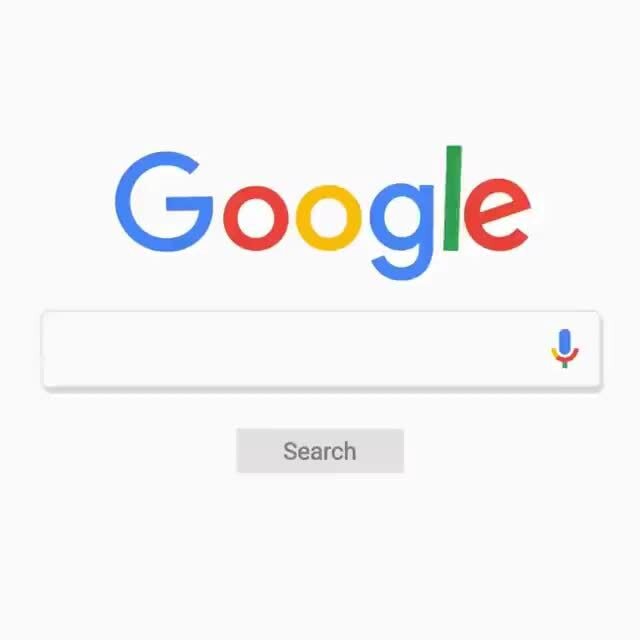This image is an up-close screenshot of the Google search page. Dominating the upper portion of the screenshot is the iconic Google logo, with its characters colored as follows: the first "G" in blue, the first "O" in red, the second "O" in yellow, the second "G" in blue, the "L" in green, and the "E" in red. Directly beneath the logo is the recognizable white search bar, which prominently features a small microphone icon to its right. This microphone icon is adorned with Google’s trademark colors of blue, red, green, and yellow. Below the search bar, there is a subtle shadow effect, giving the search bar a slightly elevated appearance. Further down, a black bar with three buttons labeled "Search" completes the interface. The rest of the screen is uncluttered, with no additional elements or text.